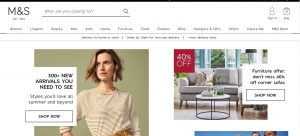The image depicts a website named "MNS," which appears to be dedicated to furniture shopping. The site's layout includes a search bar positioned slightly to the left at the top, with placeholder text that reads "What are you looking for?" Although the text on the website is generally unclear and some words are unreadable, a series of horizontal tabs are visible on the right side, allowing users to navigate through different sections. 

In the bottom left corner of the image, there is a picture of a woman wearing a brown jersey. She is positioned in front of a dark red background, facing towards the camera, but her head is turned to the left. Accompanying this image is text that reads, "All the new material you need to see," followed by a call to action to "Shop Now."

To the left of the woman, within the same image, there is a glimpse of a room that features a gray couch and a round table with a black circular stand. The room's background is predominantly dark red, comprising approximately 40% of the backdrop. Another piece of text in the scene encourages users to "Shop More."

Overall, the website "MNS" promotes various furniture items and seems to offer a range of materials and products, as indicated by the accompanying texts and visuals.